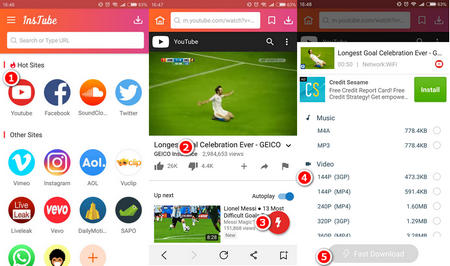In the center of the screen, there is a prominent "YouTube" label, beneath which is an image of a man kneeling on a large, vibrantly green soccer field with white boundary lines. He is dressed in a short-sleeved white shirt and white shorts, with his arms extended outward by his sides. Below the man, the text reads "Longest Celebration Ever," partially obscured by a red circle containing the number 2.

Adjacent to this, another video clip displays a man kicking a soccer ball to the right, identified as Lionel Messi. The accompanying text reads "13 Most Difficult Goals," with a red circle containing the number 3 next to it, and a red circle further right, marked with a white lightning bolt icon inside it.

In the top left corner of the screen, the heading "INS2" is seen, followed by a search bar. Below are various quick-access links, starting with "Hot Sites" and followed by: "YouTube" (with a red circle containing the number 1 to its left), "F" for Facebook, "SoundCloud," "Twitter," "Other Sites," "Vimeo," "Instagram," and "AOL." The subsequent line lists: "Lively," "Vivo," and "Daily Motion." At the bottom, there is a green circle featuring a white phone icon.